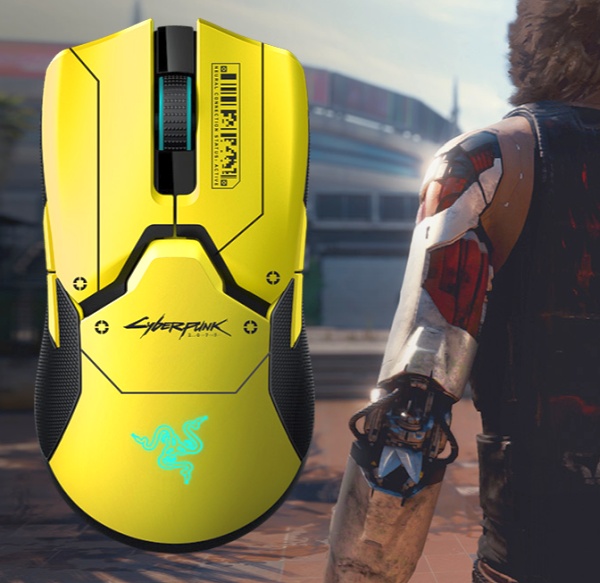The image prominently features a vivid, school bus yellow, video game-themed computer mouse occupying the entire left side. This Razer Naga mouse, adorned with black edges and rubber grips on each side, showcases a "Cyberpunk" inscription across its center in a sleek black font. The mouse is detailed with robotic-like panels, a black scroll wheel with dark green borders, and at the bottom, a glowing green triangular snake logo, emblematic of Razer. Behind and to the right of the mouse, the backdrop is a screenshot from a cyberpunk video game, partially obscured, yet vivid. The visible side shows a male character with medium length brown hair, clad in a black sleeveless shirt and dark pants. His left arm is notably robotic, displaying a polished silver surface with black tubes and red highlights near the elbow. His figure stands against the blurred impression of towering city buildings.